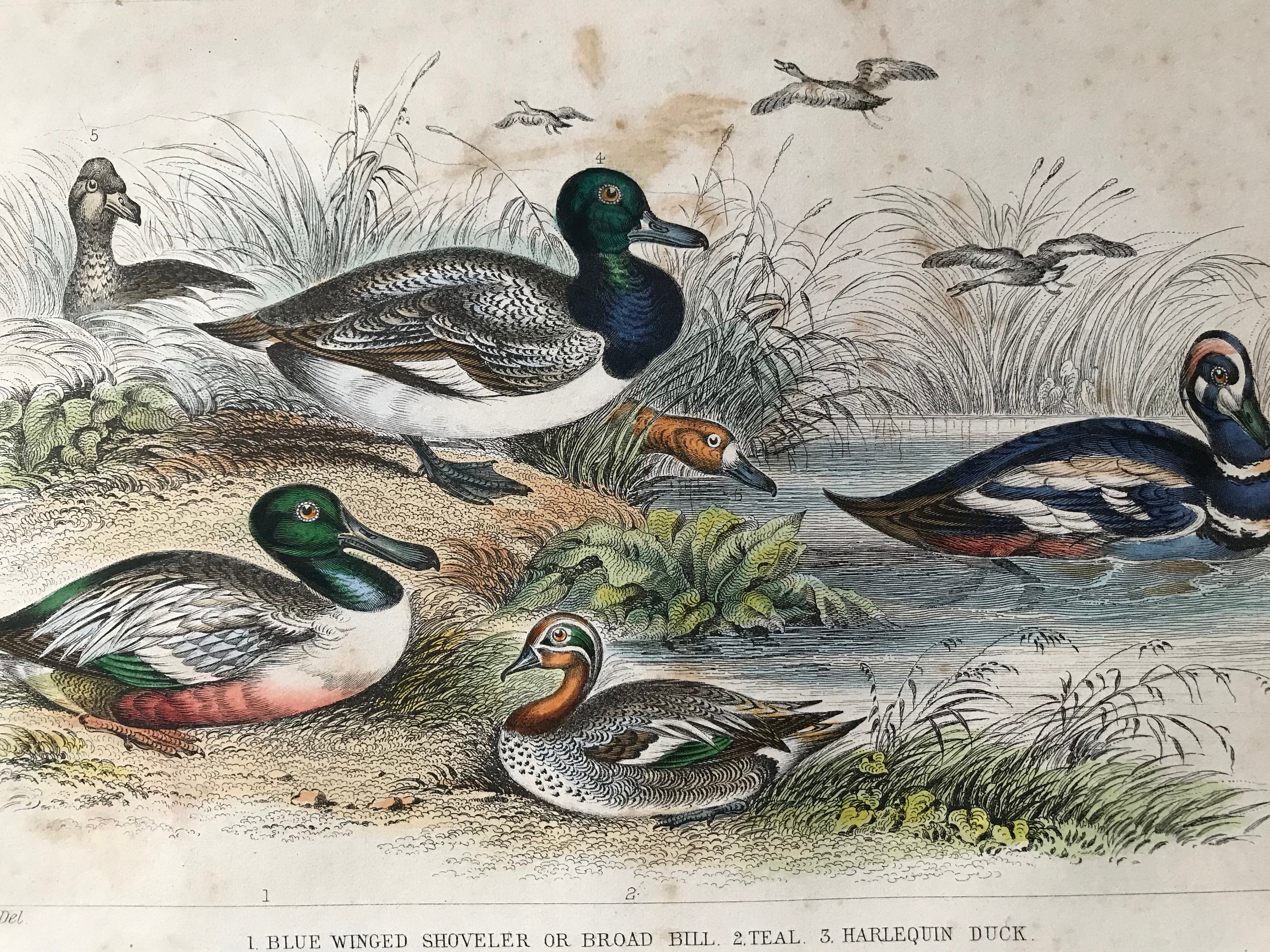This is a detailed illustration of various North American waterfowl, possibly inspired by Audubon, showcasing both flying and stationary ducks against a beige background. At the bottom of the illustration, three ducks are labeled: Number one, the blue-winged shoveler or broadbill; number two, the teal; and number three, the harlequin duck. 

At the top, a distinct black and white duck with a black head, white cheeks, and a gray beak pokes its head up. Surrounding this duck are two black and white ducks flying southward, with a smaller duck diving towards the water and the grouped ducks. Tall black and white plants frame the scene.

The central focus includes intricate details of each bird. One key duck close to the water has a brown head, a blue beak, and various shades of gray feathers on its back and neck. In the water, an elaborate duck showcases a blue crown, dark green beak, brown spots on its face, and a mix of blue, white, and red on its body. 

To the lower left, two ducks stand out: one with a blue head, gray-to-green feathers, yellow base, and orange feet; and another with an orange neck, blue beak, blue spots around the eyes, and multifaceted gray, brown, white, and green wings. Above them, another duck has gray and brown accented feathers, a white underside, gray feet, a neck fading from blue to light green, a dark green head, orange eyes, and a blue beak.

The labels and detailed descriptions emphasize the varied coloring and intricate feather patterns, making this illustration both informative and visually captivating.